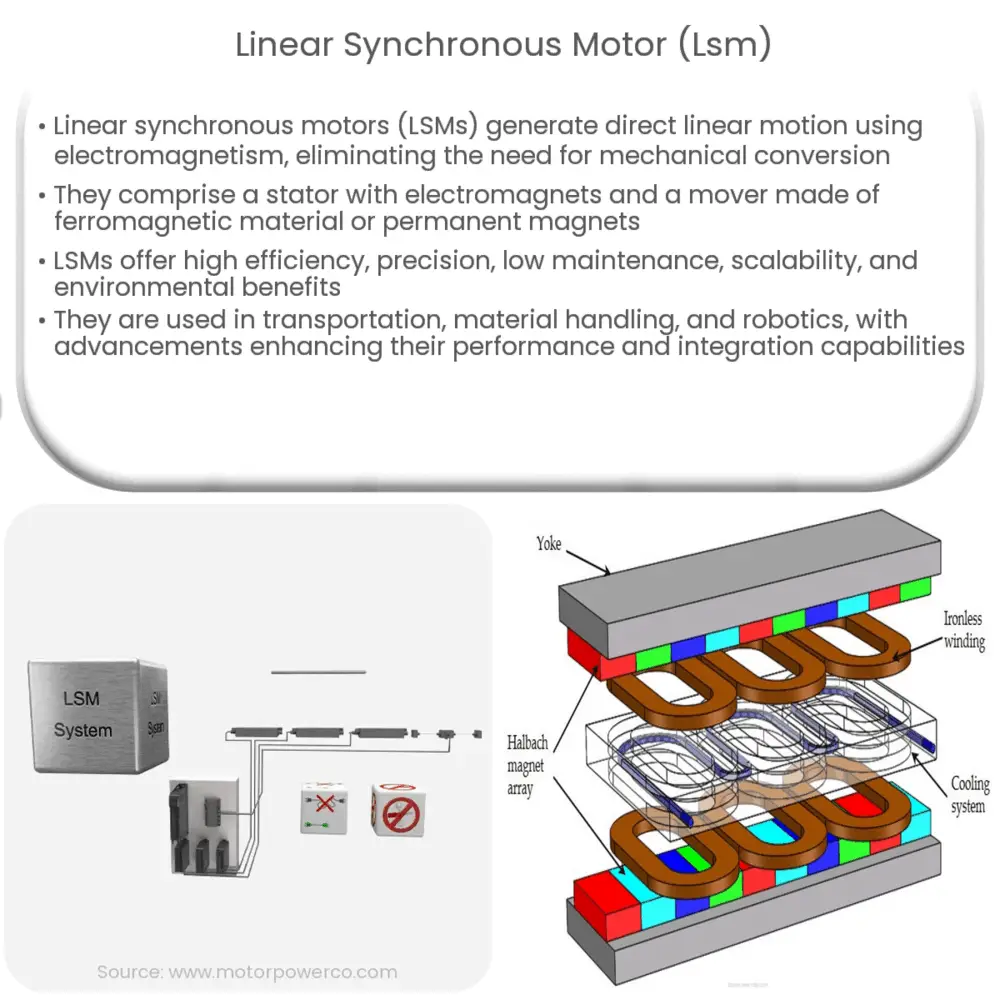The image showcases an infographic detailing a Linear Synchronous Motor (LSM). At the top center, there is a heading in gray text reading "Linear Synchronous Motor (LSM)." Below the heading, there is a bulleted list of four items, also in gray text, with an accompanying faint gray border surrounding the list. The text explains that Linear Synchronous Motors (LSMs) generate direct linear motion using electromagnetism, eliminating the need for mechanical conversion. They consist of a stator with electromagnets and a mover made of ferromagnetic material or permanent magnets. LSMs offer high efficiency, precision, low maintenance, scalability, and environmental benefits. They are utilized in transportation, material handling, and robotics, with advancements enhancing their performance and integration capabilities.

Beneath the text, on the left side of the image, there is a light gray rounded square containing a detailed illustration of an LSM system. The illustration is predominantly gray and shows machinery or circuit components labeled in black text. It includes switches connected to other electronic items and two white cube-like structures at the lower right. There are panels colored gray and coils in brown, with each part clearly labeled in black text. Additionally, the diagram features smaller elements like a red X in one box and a circle with a line through it in another, marking specific parts of the system. The entire composition uses a combination of colors and labels to visually explain the structure and function of the LSM.